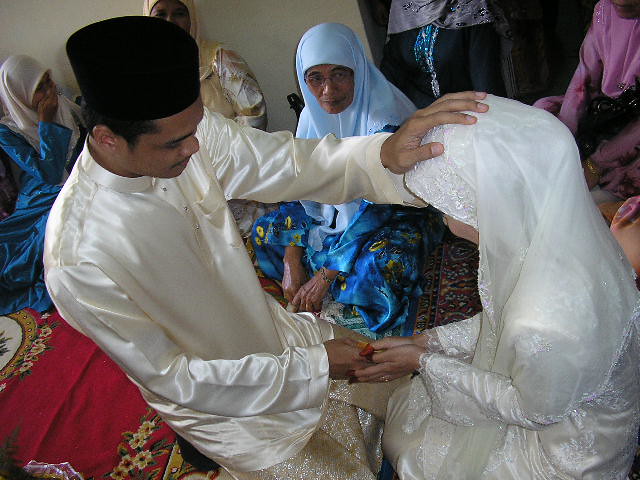The image is a vibrant color photograph that captures a solemn, intimate moment between a man and a woman at the center of an indoor setting. The foreground presents the man and woman kneeling, both with their heads bowed. The man is dressed in a champagne-colored satin long-sleeved top and pants, with a black cap atop his head, suggestive of a ceremonial role, possibly a priest. He rests one hand gently on the woman's head, while she holds his other hand in both of hers. The woman is adorned in a white veil and a long-sleeved white dress, reinforcing the ceremonial nature of the scene.

Surrounding the central figures, several other individuals are attentively witnessing the moment. Directly behind the couple, a woman is wearing a white veil and a blue long-sleeved outfit, covering her mouth with her hand as if in emotional reaction. Another woman is resplendent in a gold outfit with a matching headdress. To the right, a woman donning a blue scarf over a dark blue dress and robes stands in contemplation. Additionally, in the corner, an individual wears a pink long-sleeved top.

The background reveals more about the setting, with a noticeable carpet on the ground and a table partially visible in the bottom left corner. This intricate social gathering, cloaked in ceremonial attire of various colors like red, yellow, green, tan, white, light blue, blue, purple, and pink, suggests a rich cultural context. The indoor scene, presumably lit by daylight, enhances the vividness of the event being photographed, capturing a serene, prayerful interaction at its core.